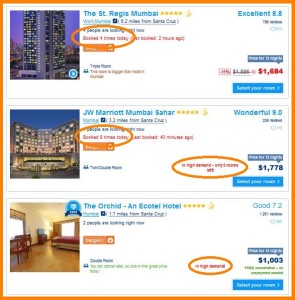The screenshot we are examining is square-shaped, bordered by a solid orange line. It contains three horizontally aligned images, stacked vertically atop one another.

The first image depicts a city scene and features a blue text overlay at the top paired with a rating of five stars. At the uppermost part of the image, there is a yellow circle with blue text that indicates the price and rating. The hotel showcased in this image is the St. Regis, with a rating described as "Excellent 8.8."

The second image also has a notable orange circle containing blue and red text, which signifies the price. Another orange circle near the price displays the value in blue. This image rates the hotel as "Wonderful 9.0" and captures the JW Marriott Mumbai.

The third and final image prominently features the Orchid hotel. Similar to the previous entries, this image includes visible text overlays and rating information.